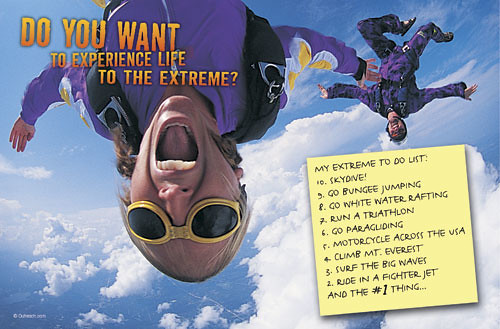In the vibrant image, two skydivers are captured mid-fall against a backdrop of a bright blue sky adorned with fluffy clouds. The scene is oriented upside-down, intensifying the exhilarating chaos. The foremost skydiver, garbed in a purple jumpsuit with black straps and a backpack, has their mouth wide open as if screaming, and they're wearing distinctive yellow goggles with black lenses. The second skydiver is visible in the background, also upside-down, with their arms stretched out and knees bent, floating in the gravity-defying moment.

The upper left corner of the image features bold, capitalized text in a gradient of yellow and orange, reading, "DO YOU WANT TO EXPERIENCE LIFE TO THE EXTREME?" The lower right corner showcases a yellow post-it note with the header, "MY EXTREME TO-DO LIST." The list itemizes thrilling activities from number 10 down to 1, including "10. Skydive, 9. Go bungee jumping, 8. Go whitewater rafting, 7. Run a triathlon, 6. Go paragliding, 5. Motorcycle across the USA, 4. Climb Mount Everest, 3. Surf the big waves, 2. Ride in a fighter jet," with the number one item intriguingly left blank, indicated by an ellipsis: "...". The cumulative elements of the image and text invite viewers into a realm of adrenaline-pumping adventures and the ultimate pursuit of life's extremes.